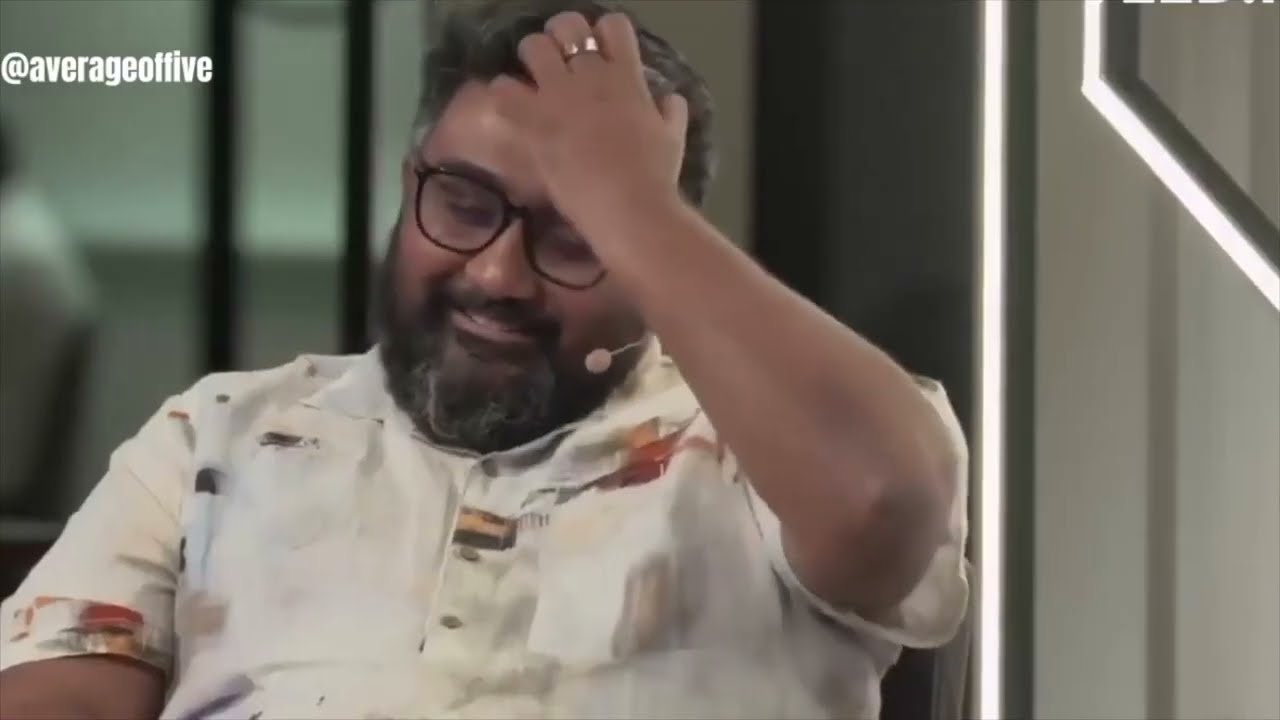In this image, a heavyset man with brown skin and dark hair is seated, positioned slightly at a diagonal. He has a thick beard flecked with gray at the chin, a mustache with some silver strands, and wears black-framed glasses. He is smiling with his eyes closed, scratching his head with his left hand, which has a ring on the middle finger. The man is wearing a short-sleeve white shirt adorned with red, brown, and black patches. A thin wire microphone with a small fuzzy ball is attached near his mouth, indicating he is speaking or preparing to speak. The background features predominantly gray, white, and light green colors with vertical black and white stripes, and blue and gray rectangles. In the upper left corner, there is white text reading "@averageoffive."